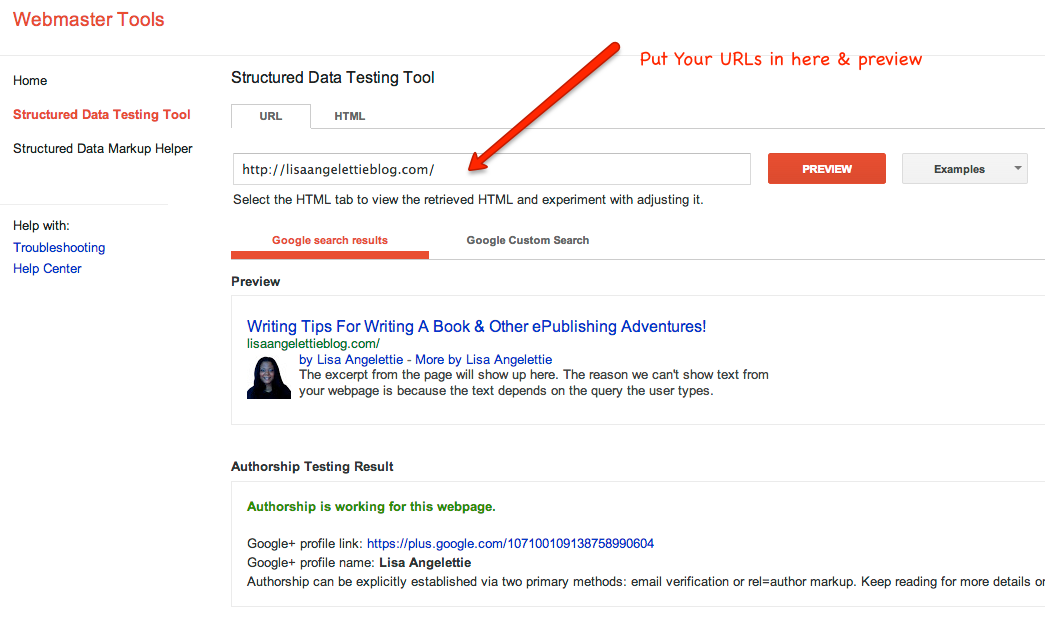A detailed screenshot caption of the Webmaster Tools interface, marked up with annotations in red:

"The screenshot displays a marked-up interface of Webmaster Tools. In the upper left-hand corner, a red font label reads 'Webmaster Tools.' 

A line divides the page into two columns. The left column features several elements starting with 'Home' at the top. Further down, a row in red font highlights the 'Structured Data Testing Tool,' followed by a row in black text that reads 'Structured Data Markup Helper.' There is a small gap before another section labeled 'Help With' in black, under which 'Troubleshooting Help Center' is displayed in blue.

The highlighted 'Structured Data Testing Tool' in the left column corresponds to the right column content. The right column begins with the 'Structured Data Testing Tool' title, under which are two interactive tabs labeled 'URL' and 'HTML.' Below these tabs, there is a large input form where users can type in a URL. To the right of this input box, a 'Preview' button is available, and even further right, a drop-down menu labeled 'Examples' can be found. Beneath this section, an instructional text advises users to select the HTML tab to view the retrieved HTML and experiment with adjusting it. 

At the bottom of the right column, two separate sections are labeled 'Google Search Results' on the left and 'Google Custom Search' on the right.

A prominent red arrow annotation points directly to the URL input area at the top of the right column, accompanied by the text 'Put your URLs in here and Preview,' guiding users on how to utilize the tool."

This caption provides a comprehensive, step-by-step description of the screenshot and its annotations, offering clarity on how the interface is structured and what the key elements are.